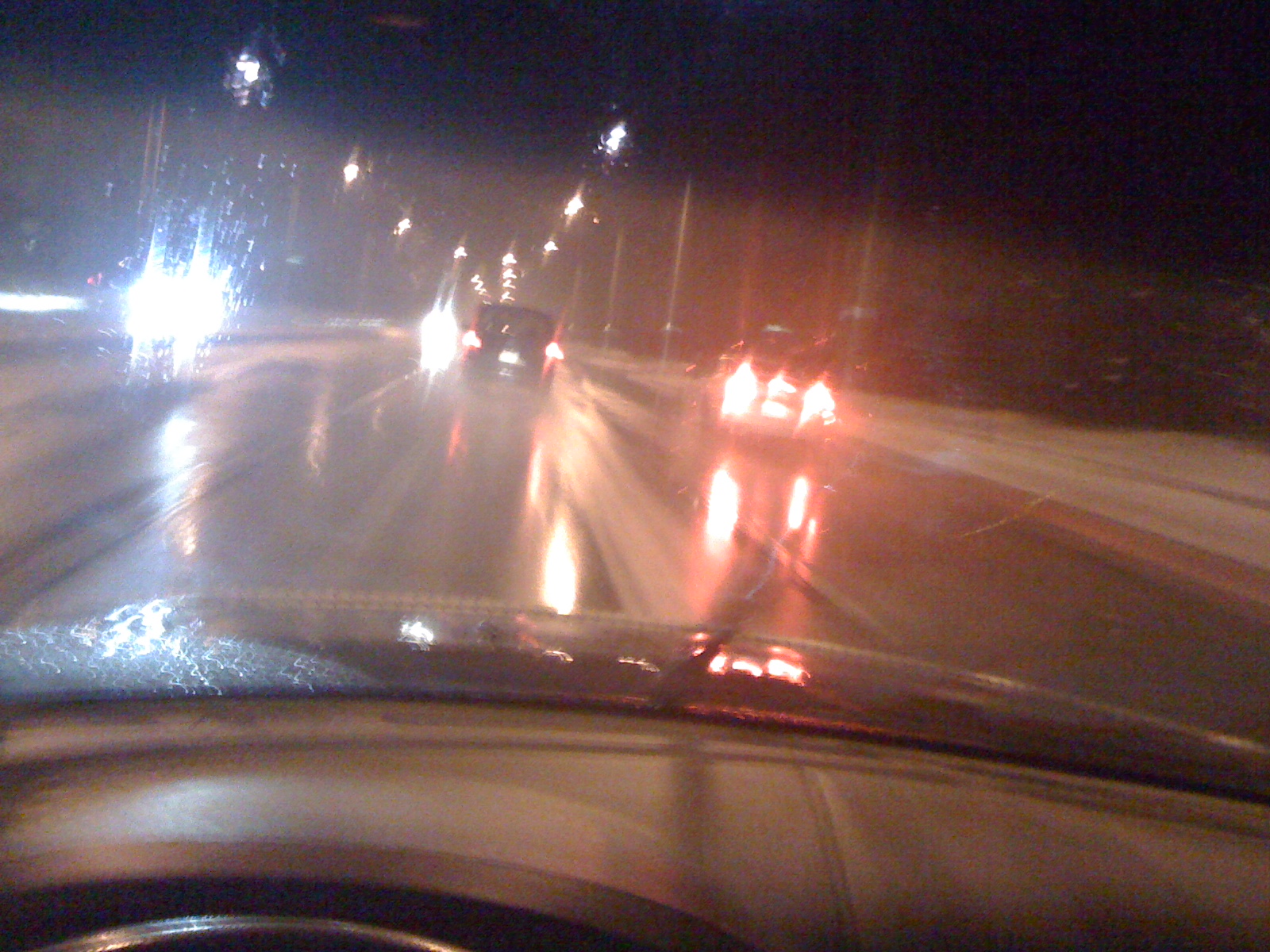A nighttime view from inside a car captures the essence of a rainy drive. The roads glisten with fresh rain, indicating it's currently showering. Raindrops speckle the windshield, which is partially cleared by the wipers—the moment captured as the wiper blade is midway across. The motion blur suggests the shot was taken while the car was moving. Two vehicles with red brake lights are ahead on this apparent four-lane highway, while two cars with blue headlights approach from the opposite direction. Numerous street lights dot the road, their glow extending far into the distance and reflecting beautifully off the car's hood, enhancing the atmospheric mood of the scene.